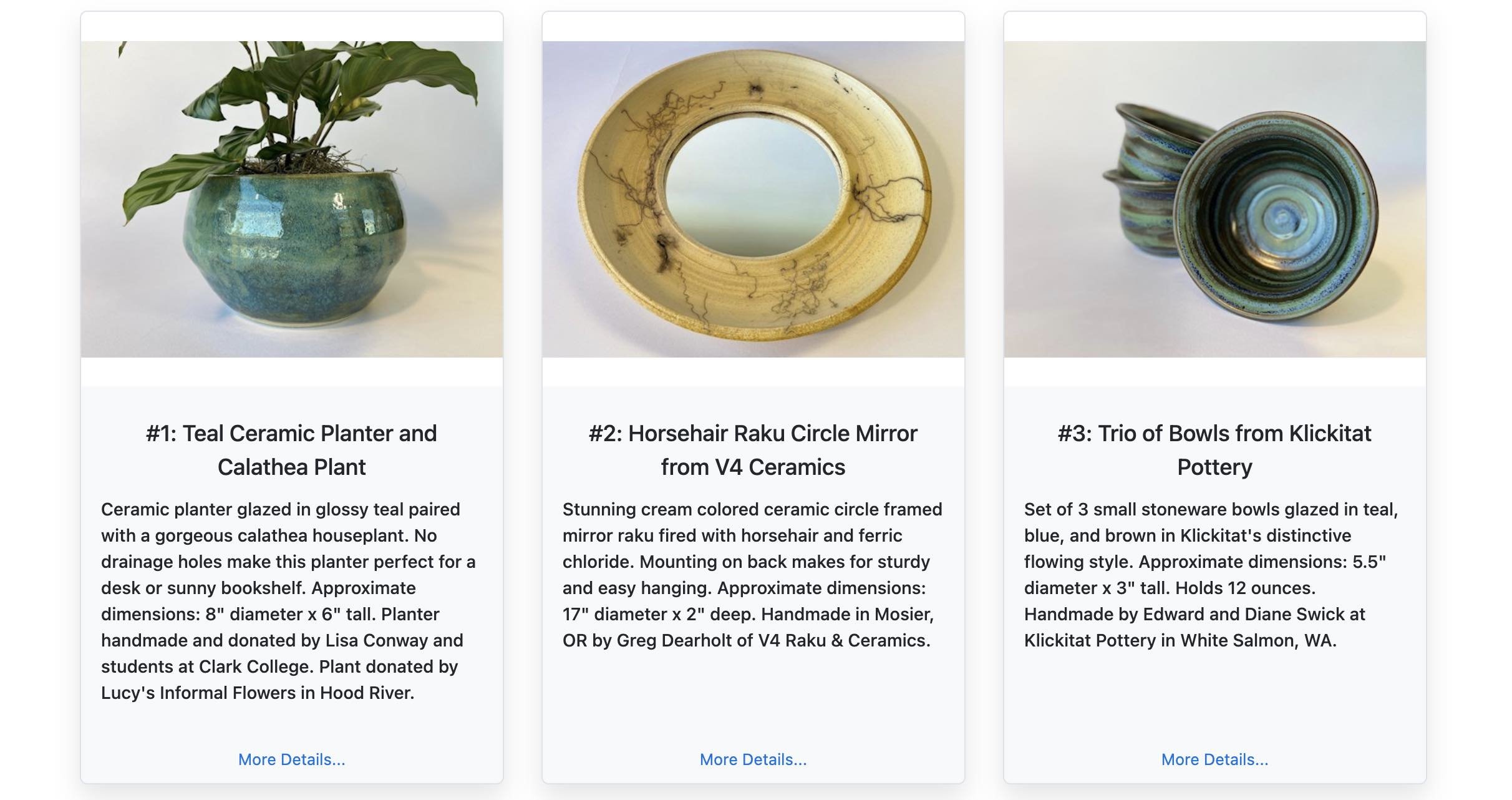The image features a triptych of color photographs, each paired with detailed descriptive text below. On the left is a "Teal Ceramic Planter" housing a lush Calathea plant, both serene and glossy. In the center, there's a "Horsehair Raku Circle Mirror" from V4 Ceramics, resembling a wide, yellow donut with intricate black streaks. To the right, a "Trio of Bowls" from Klickitat Pottery displays a set with two bowls stacked and a third on its side, revealing a swirling blue interior. Each image is uniformly sized, with black text on a white background beneath them, and a consistent blue hyperlink for "more details..." at the bottom of each section. The composition blends photographic realism with graphic design elements.